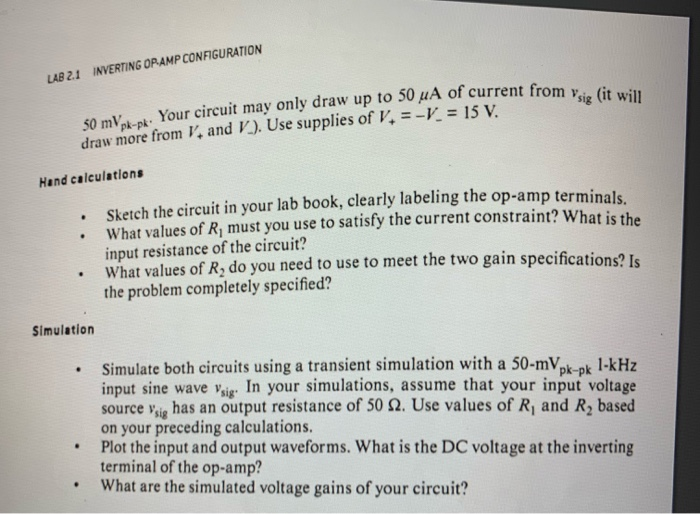This is a black-and-white image of a page from what appears to be an instructional textbook. The page is oriented horizontally, with the top edge visible at the upper right corner, extending diagonally down and to the left, and then off the image at the bottom right, giving it a slightly curved appearance. The left edge of the visible part of the page shows the header "Lab 2.1: Inverting OP AMP Configuration" in bold black text. Below this header are two sentences of printed text, containing what looks like calculations and symbols.

Following this, there's a bold heading titled "Hand Calculations," under which there are three bullet points with corresponding descriptive sentences. These bullets and descriptions formulate questions about sketching circuits, labeling operational amplifier terminals, determining resistor values to meet current constraints, and finding the input resistance of the circuit.

Further down, there's another bold heading labeled "Simulation." This section also contains three bullet points, with lines of text describing the simulation tasks. The first bullet point spans four lines, the second two lines, and the third only one line. The image cuts off the bottom left corner, partially obscuring some of the text in the simulation section.

Overall, the content suggests the page is likely related to a mathematics or computer science discipline, focusing specifically on operational amplifier configurations and their calculations and simulations.